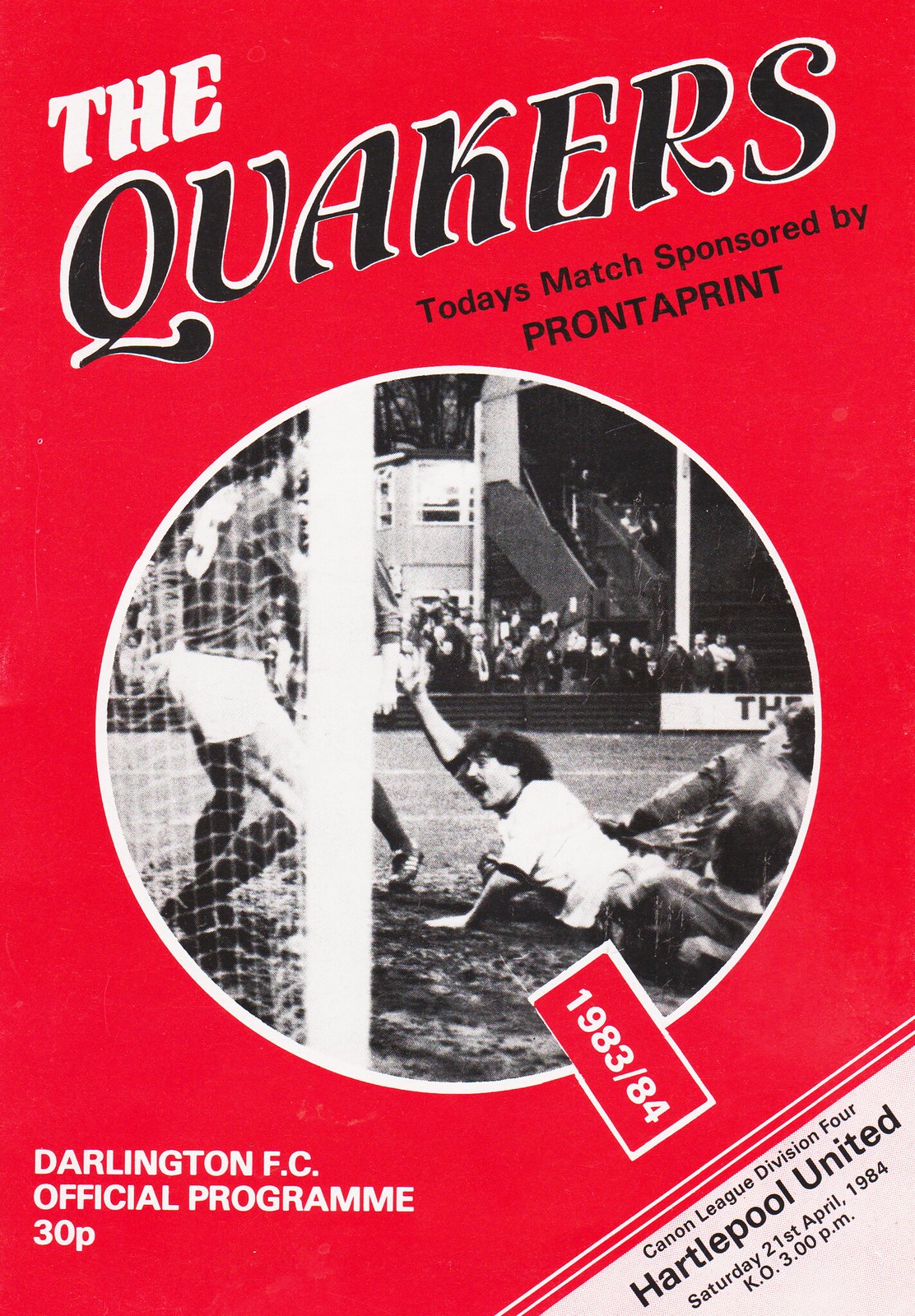The image is a vintage brochure for a soccer match, featuring a bright red background with a circular black-and-white photograph in the center. The photograph depicts a scene from a soccer game, showing several players and a goal net with a goalkeeper. At the top of the brochure, the title "The Quakers" is prominently displayed in stylized black and white text. Right below, it mentions, "Today's match sponsored by Prontoprint." At the bottom of the brochure, it specifies "Darlington FC Official Program" along with the price "30p" and the season "1983-84." Additionally, on the bottom right corner, the details read "Canon League Division 4, Hartlepool United, Saturday 21st April 1984, KO 3 p.m."